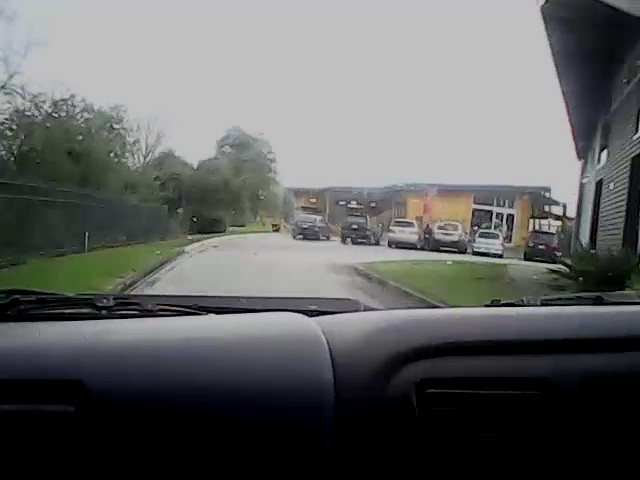In this real-life photograph captured from the inside of a vehicle, the bottom edge of the image displays the top part of the car's dashboard and partially visible windshield wipers, obscured by heavy shadows. Beyond the windshield, the viewer is presented with a scene of a narrow roadway flanked by greenery, including a mowed lawn on the left and a fence with blurry, pixelated trees in the background. The image quality is low resolution and seems to have been taken on a cloudy day, evidenced by the overcast sky that appears as a grayish-white color. On the right side of the image, there is a building partially in view, showing its front facade and a protruding roof providing shade. Dominating the center foreground is a modern yellow building characterized by a slanted roof and a large window. In front of the building, about five cars are parked, indicating that the vehicle from which the photo was taken is driving towards this area.